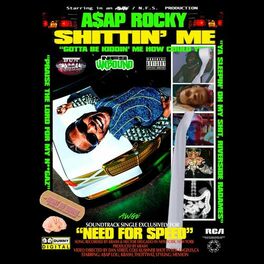The image is a square, likely a poster or an album cover, with a solid black background. At the very top, there are small, unreadable white prints followed by bright neon green bold text that reads "A$AP Rocky," with the S stylized as a dollar sign. Directly beneath, in bold yellow letters, it says "SHITTIN' ME" in all caps. Centered in the middle of the composition is a sideways photograph of A$AP Rocky, an African American man, wearing black sunglasses and a blue shirt with black and white sleeves. On the right side of the album cover, there is a vertical arrangement of five smaller, hard-to-see images, including one resembling an X-ray of a spine and abdomen. Towards the bottom, bold yellow text in quotation marks says "NEED FOR SPEED." The lower right corner of the cover features a white RCA symbol, and the background contains faint additional words in various bright colors that are difficult to discern, adding to the layered and complex design.